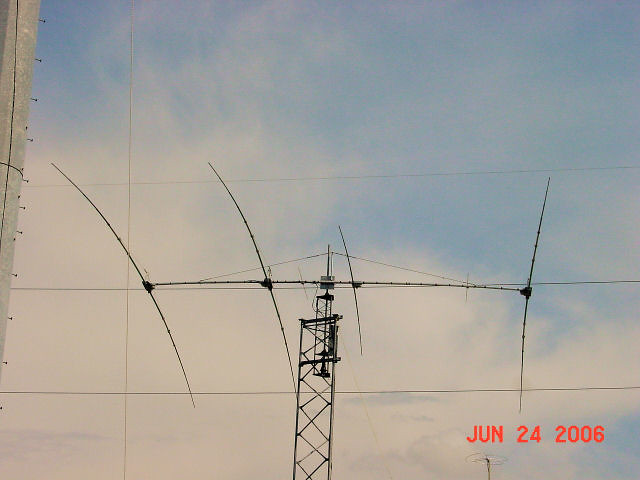The photograph, taken on June 24, 2006, features a bright, partly cloudy sky with wispy white clouds against a blue background. The timestamp in the bottom right-hand corner is clearly marked in orange font. The central focus is a metal tower supporting power lines, situated prominently in the middle of the image. This steel structure has various metal rods branching off, connecting multiple strings of power lines above and below. Mounted at the top of the tower is a small metal deck, likely meant for maintenance personnel. On the left side of the photograph, a grayish steel pole is visible with climbing pegs attached, though only the lower half of this pole is in the frame. The photograph captures both the intricate details of the electrical infrastructure and the serene outdoor environment.